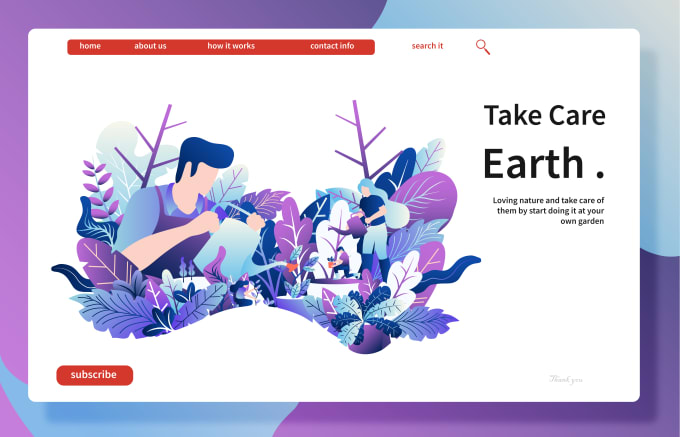"Screenshot of a website with a vibrant, multicolored frame. The left and top-left borders of the screen are purple, while the bottom and right sides are split between gray and purple. The top-right section is a grayish-blue hue.

Centered on the screen is a white block with red tabs in the top-left corner, featuring the words 'Home,' 'About Us,' 'How It Works,' and 'Contact Info' in white text. Adjacent to these, a red 'Search It' button with a red magnifying glass icon lies to the right.

Below the tabs, the webpage showcases an image of individuals tending to a garden. Two people are seen watering plants with watering cans, and a third person in the background appears ready to plant a seedling. The overall color scheme of the image includes shades of grayish-green, blue, and purple. To the right of the garden scene, the phrase 'Take Care Earth' is prominently displayed. In the bottom-left corner of the screen, a red 'Subscribe' button is visible."